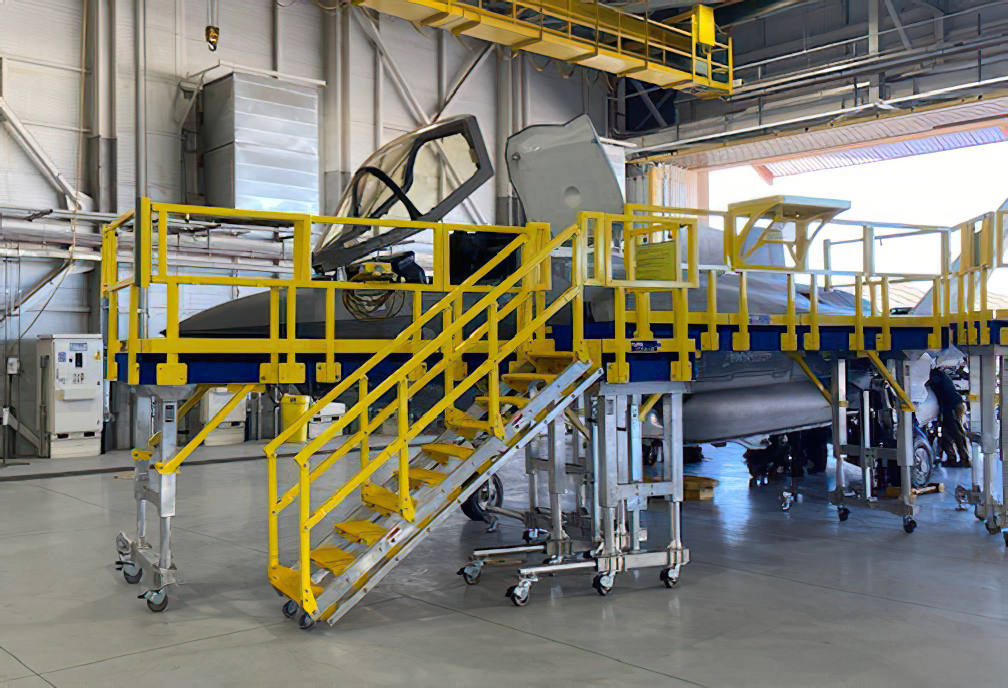This is a realistic, color photograph taken in a spacious, industrial airport hangar with a very metallic, industrial aesthetic. The hangar features numerous metallic silver finishes and scaffolding, with the floor covered in gray tile. Yellow and blue scaffolding structures are prominently displayed, with some yellow scaffolding extending toward the ceiling and more mixed with blue in the foreground. A movable, wheeled staircase is attached to the scaffolding, which surrounds a gray aircraft that resembles a private jet. The jet's front window is designed to pop open, as seen on some jet planes. People are visible working on the aircraft, including one individual in the bottom right corner, who appears to be inspecting or fixing the back of the plane. This person is wearing a blue top and dark brown khaki pants. There is also a concrete brown box beneath the jet. The hangar's metallic elements, combined with the industrial scaffolding and tools, contribute to the overall functional and utilitarian feel of the space.